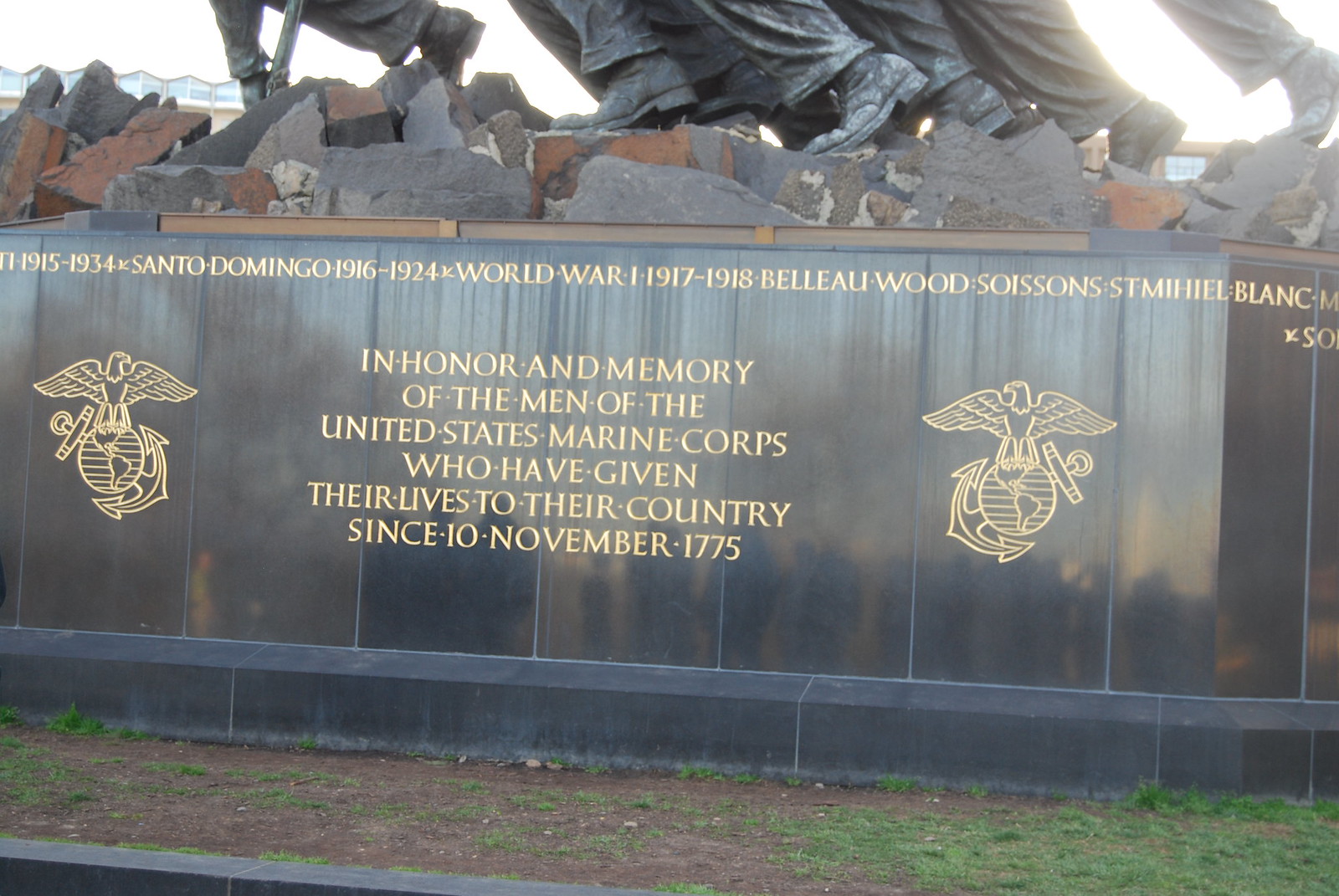This is a horizontally aligned rectangular picture of a stone monument with a tall base, approximately four to five feet in height, featuring an engraved plaque. The base of the statue is a blend of brown and gold hues, with gold print detailing significant historical dates and locations: "Santo Domingo, 1916 to 1924," "World War I, 1917 to 1918," and names such as "Belleau Wood" and "Soissons," along with other entries in another language.

The central focus of the plaque is an inscription in honor of the fallen soldiers of the United States Marine Corps, which reads, "In honor and memory of the men of the United States Marine Corps who have given their lives to their country since 10 November, 1775." Flanking this inscription are two symbols depicting bald eagles with wings spread, perched atop globes with anchors through them, likely representing the Marine Corps emblem.

Above the plaque, the statue features a collection of rough rocks in gray and a few red hues, upon which rest multiple stone legs and booted feet. Visible at the very top of the image is a sliver of sky, appearing white, while the foreground includes a mix of dirt and grass in front of the monument's base.